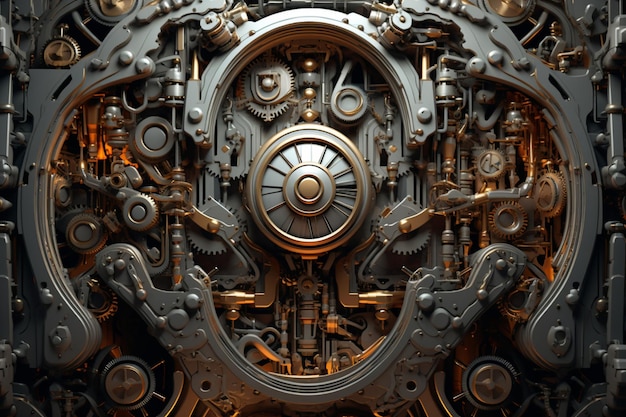This image features a detailed, computer-generated close-up of an intricate machine mechanism, devoid of a background or borders, giving it a square, stand-alone appearance. Predominantly gray, with areas highlighted by coppery tones and orange lights, the composition is a complex array of interlocking gears and mechanical parts. Central to the image, towards the top, is a white number 6 adorned with a gold band encircling the upper part. Flanking either side at the bottom are two semicircular strips of dark silver, resembling pewter. With a myriad of circles, gadgets, and gears throughout, the overall impression is that of a futuristic or fantastical device, evoking the inner workings of a time machine. The purpose of the machine remains ambiguous, adding an air of mystery to its elaborate design.